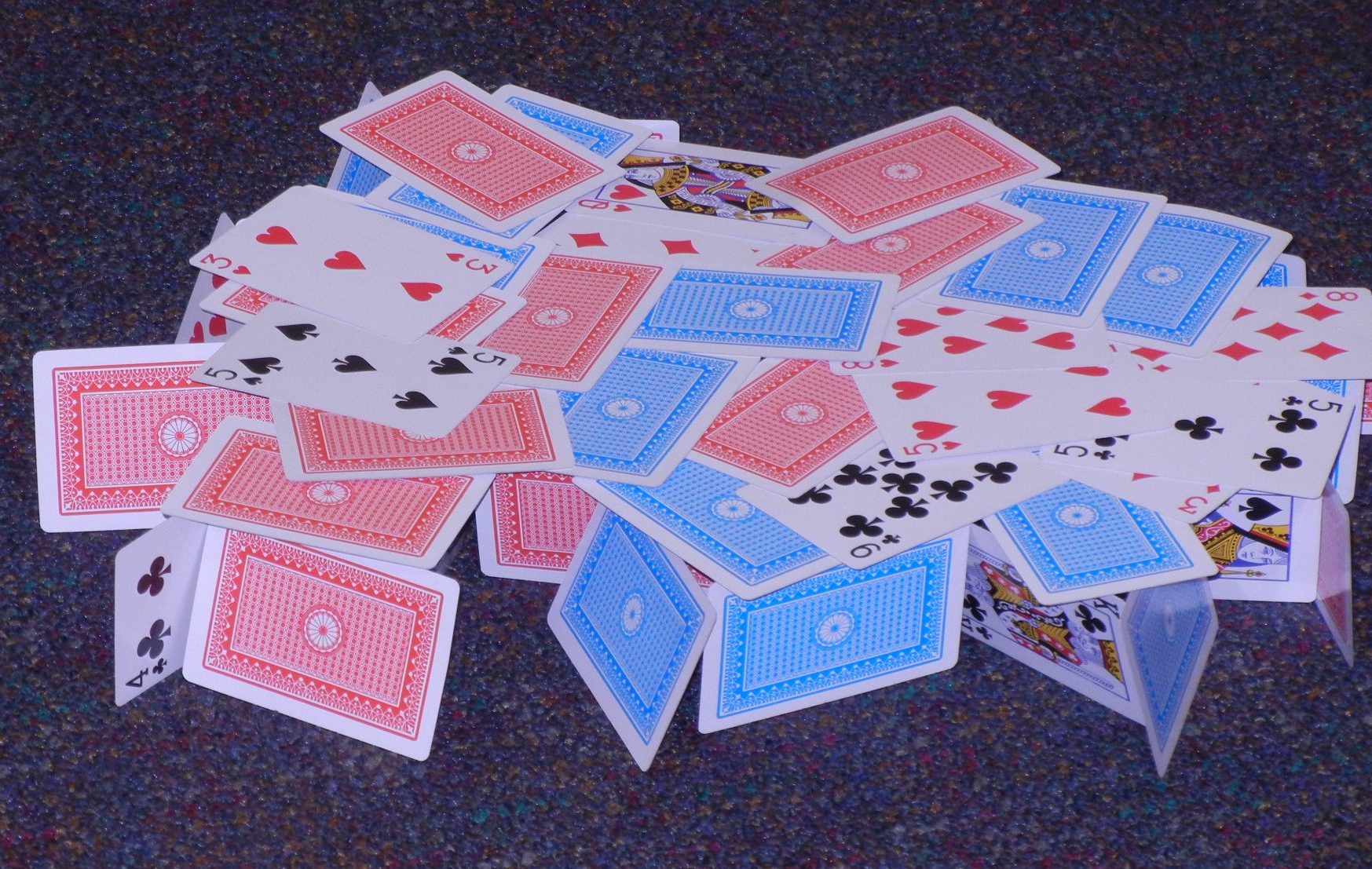This is a color photograph featuring a scattered arrangement of playing cards on a textured blue or dark gray carpeted background. The cards are fanned out in a somewhat haphazard manner. Some card backs are blue, while others are red. Several cards are facing up, displaying a variety of values and suits including the 9 of Clubs, King of Clubs, Queen of Spades, 5 of Clubs, 5 of Hearts, 5 of Spades, 3 of Hearts, and 4 of Clubs. The mix of face-up and face-down cards, combined with the contrasting colors of the card backs, creates a visually engaging and dynamic scene.